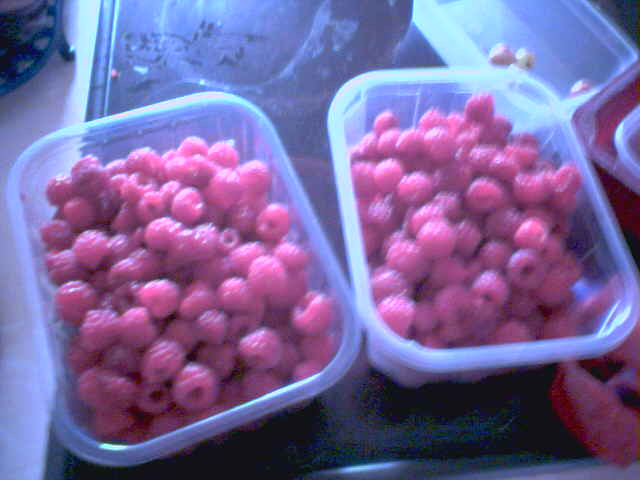This color photograph presents a close-up view of two square plastic punnets filled with red raspberries, placed side by side on a dark-colored table. The slightly out-of-focus and desaturated image gives the scene a muted and dreamy appearance. The containers, made of clear and slightly opaque plastic, are rectangular with rounded edges, each filled randomly with ripe raspberries displaying their characteristic lumpy texture and stem indentations. Just to the upper right of the punnets, an additional container lid is visible, while at the lower right-hand corner, there's another container with a few raspberries, alongside a red and white striped object. The dark table beneath seems to reflect light around the edges of the containers, and in the upper left-hand corner, a roundish blue metal object, possibly a chair or stand, adds to the composition. On the left, a portion of a beige floor is minimally seen, providing a contrasting backdrop to the dark table.